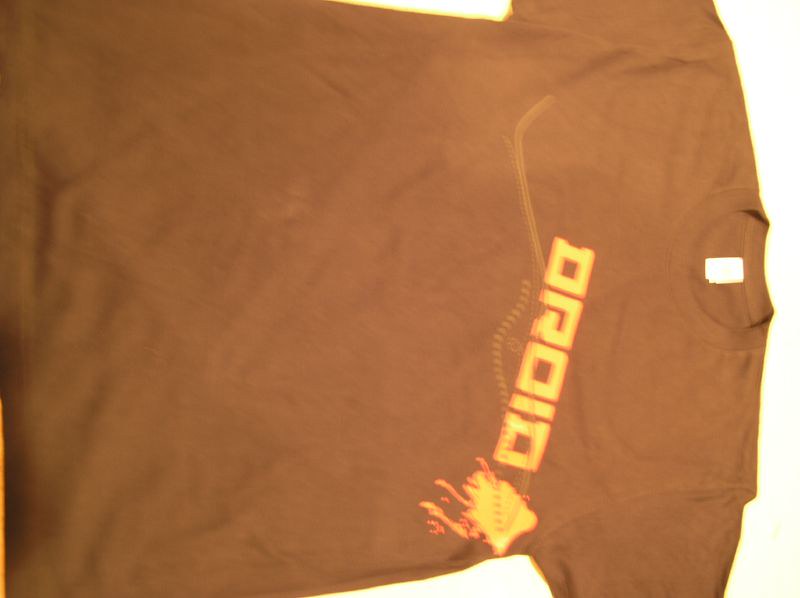This image portrays a somewhat wrinkled, brown t-shirt turned sideways, such that the collar is oriented towards the right side of the photo. A noticeable white tag is present, although any writing on it, such as the size or brand, is obfuscated by a light glare. The t-shirt appears approximately seven inches long vertically and nine inches wide horizontally. The main feature is an orange and yellow text with block letters that is difficult to decipher but seems to spell out a sequence such as "D R O I" or "O R O I O." The text is accompanied by a small yellow rectangle outlined in orange, with what appears to be a fire symbol or flames extending from it. The overall color perception might be influenced by the lighting in the image, lending to some ambiguity.